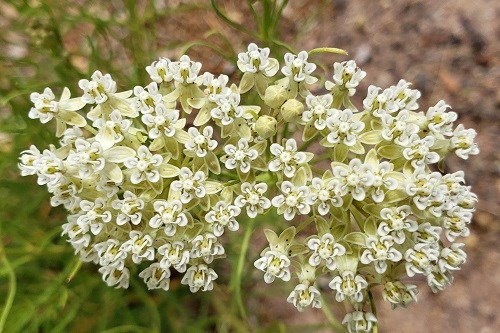This is an outdoor photograph featuring a close-up, overhead shot of a dense cluster of white flowers at the center. Each small flower has five petals, and the plant displays numerous blossoms, giving it a lush and almost entirely white appearance. You can also see some light green bulbs that have not yet bloomed. The background is distinctly divided: the right side is a lighter brown dirt area with pebbles, while the left side is primarily green grass with some plant leaves. The upper part of the background appears a bit blurry, emphasizing the clarity and detail of the blooming flowers in the center. The green stems and leaves beneath the flowers add a contrasting texture to the image.